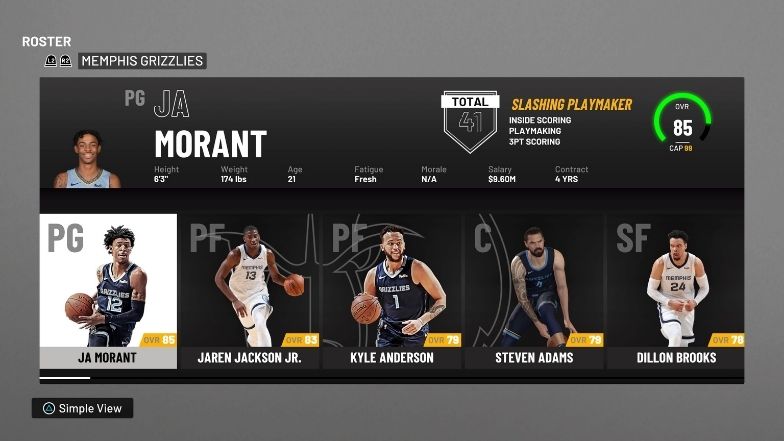This image captures a player profile screen from the NBA 2K series video game, specifically spotlighting the player Ja Morant. The backdrop is a sleek grey. Positioned at the top-left corner is the word "Roster" displayed prominently in bold white text. Beneath this are two small black icons, adjacent to a black rectangular box that boldly states "Memphis Grizzlies" in white letters.

In the center of the grey background lies a large black rectangle. In the top-left corner of this rectangle is a photo of Ja Morant. To its right, it indicates his position as "PG" (Point Guard) and lists his name, "Ja Morant." At the top-right of the black rectangle, a small icon denotes "Total 41." Adjacent to this, the words "Slashing Playmaker" appear in bold orange, next to a performance gauge reading 85.

Below this section are five player thumbnails, each annotated with their respective names at the bottom and their positions indicated in the top-left corners. Finally, at the bottom-left of the grey box, there is a button labeled "Simple View."